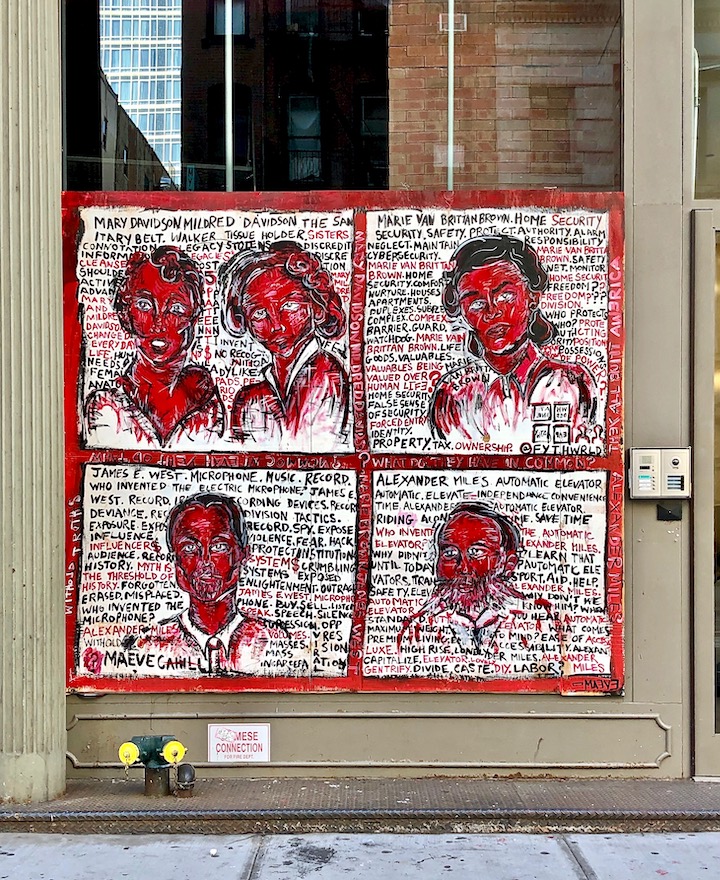The image depicts an urban scene viewed from a sidewalk, capturing part of a gray concrete walkway with scattered leaves and stains. The main focus is a large window on an adjacent building, framed on the sides with light gray borders. A metal walkway is present in front of the window, behind which is a sectioned sidewalk. The window has a clear upper portion revealing urban buildings, including a brick structure and a glass-fronted building, with darker buildings in the background.

Attached to the bottom part of this window or door is a poster divided into four quadrants, bordered by a red outline. Each quadrant features a white background with rows of text behind images of people. The top left panel shows two women with red faces and black hair, the top right panel depicts a single woman with similar features, and both bottom panels showcase men with red faces, black hair, and white shirts shaded in red. The text on each panel and the red borders separating them provides information about these individuals.

Additionally, a small cup containing yellow flowers is seen near the door, which also has some form of tan or beige lock system and a sign with names and achievements, seemingly paying homage to notable individuals, possibly African-American inventors, including references to inventors of the microphone.